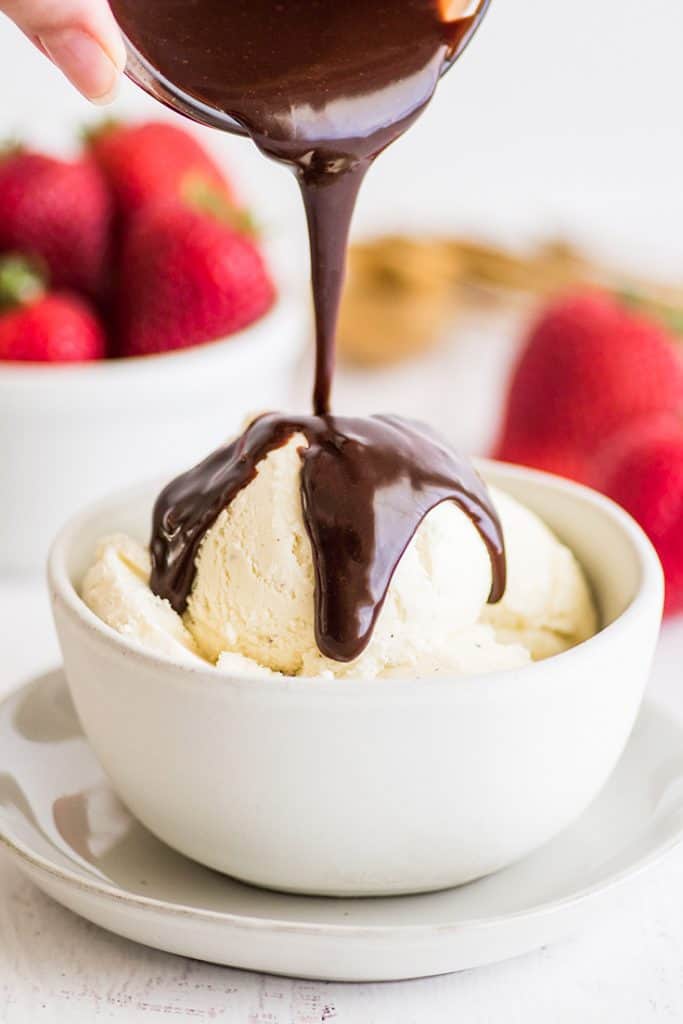A close-up image captures a delectable scene of a vanilla ice cream sundae being prepared. The ice cream is nestled in a small, white bowl set on a matching saucer. A thick, chocolate mousse is being poured over it from a glass container, with only a thumb and finger visible as they hold the container. The chocolate sauce cascades onto the ice cream, creating a mouth-watering visual. In the blurred background, there's a collection of fresh strawberries - two directly to the back right of the ice cream and a small, similar white bowl to the back left overflowing with strawberries, their green tops still intact. The table beneath the setup appears brown with light markings. A faint yellow blur, possibly a banana, is also faintly visible in the distant background, adding to the summery feel of this enticing ice cream scene.